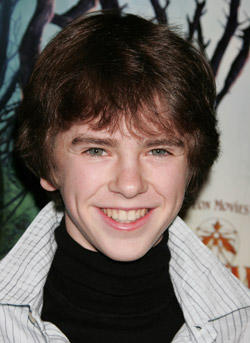The photograph features a close-up headshot of a smiling younger man with light-colored eyes, possibly blue or green. His medium-length brown hair, styled in a somewhat wavy and mop-like bowl cut, falls near his eyes and forehead. He is dressed in a black turtleneck shirt layered under a white, grey-striped button-up shirt, with the top buttons undone. His smile reveals the top half of his large white teeth. Behind him, the background is predominantly white but adorned with a brown painted tree without leaves. To the right, there are indistinct orange words, with "movies" being the only legible term. The overall vibe of the image suggests a vintage touch, inferred from the man's attire and hairstyle.